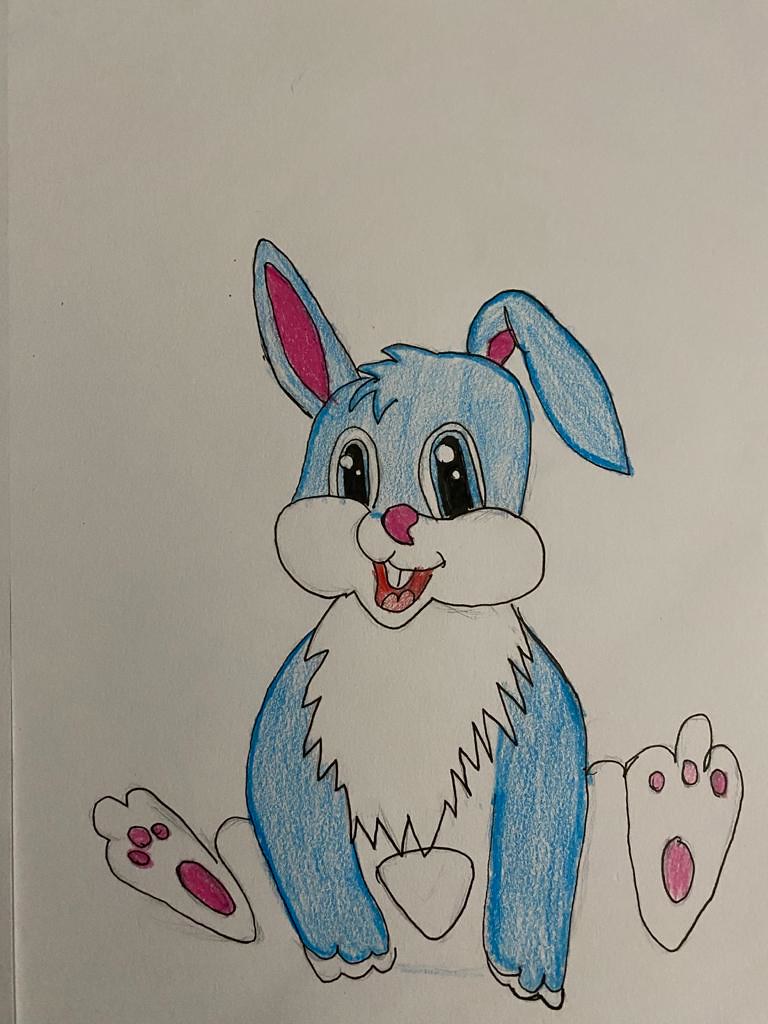The image depicts a pencil-colored bunny facing the camera. The bunny sits with its arms lying between its legs, showcasing a charming combination of colors. Notably, the right ear is curled over while the left ear stands upright, with pink centers. The bunny’s head is predominantly blue, with a tuft of hair on top. Its eyes are large and unique, being blue with black pupils and white highlights. The bunny’s nose and mouth area are pink, while its cheeks are white, contrasting the otherwise blue face. The bunny’s mouth is slightly open, revealing its front two teeth. It boasts thick fur around its neck and the tops of its arms are also blue. The back legs, lifted and showing the pink pads on the soles, add to the cuteness of the drawing. The background is white, and the image rests on what appears to be gray paper, indicating that it's possibly part of a well-done coloring page. Overall, the detailed and cohesive rendering highlights the bunny’s playful and endearing appearance.